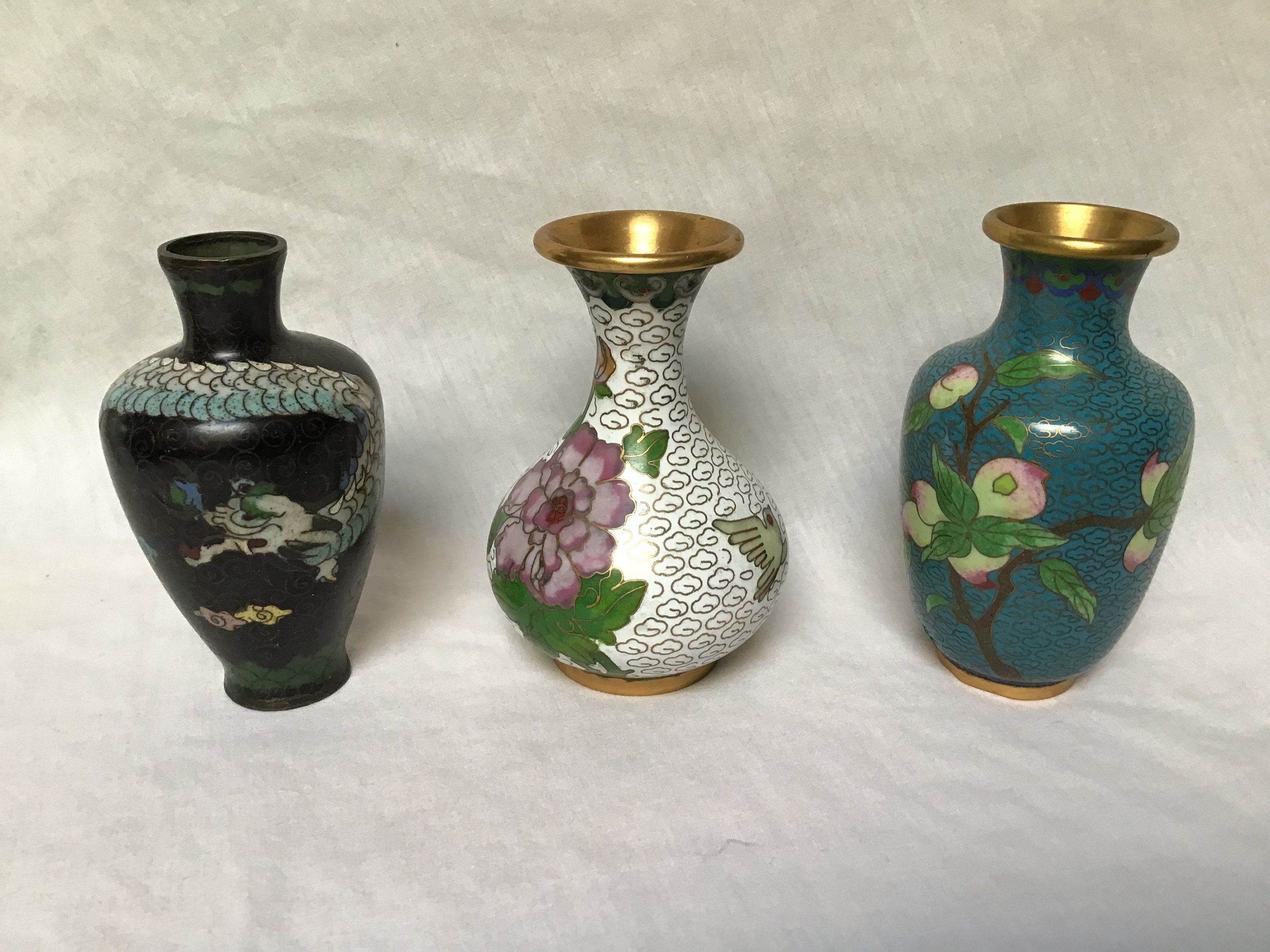This professional photograph showcases three ornate antique vases, meticulously displayed against a backdrop of curved gray fabric or canvas. Each vase is of the same height but distinct in design. 

On the left is a black vase adorned with an eastern-style dragon featuring light blue scales. The base of this vase transitions into green with a hint of yellow. Gold trims add a touch of elegance at both the bottom and top.

In the middle stands a white vase with golden cloud patterns. The centerpiece is a large purplish-pink flower with detailed petals and green leaves, accompanied by the partial view of a small winged bird. This vase also has gold accents along the rim and bottom, and intriguingly, the inside appears to be coated with a metallic finish.

The vase on the right is predominantly dark blue and features a single branch adorned with peach-colored flowers—white on one side and pink on the other. The blossoms, possibly dogwood, are complemented by green leaves. Similar to the middle vase, it also has gold trims along the top and bottom.

All three vases sit gracefully on a cloth-draped table that continues into the backdrop, creating a cohesive and elegant display setting.